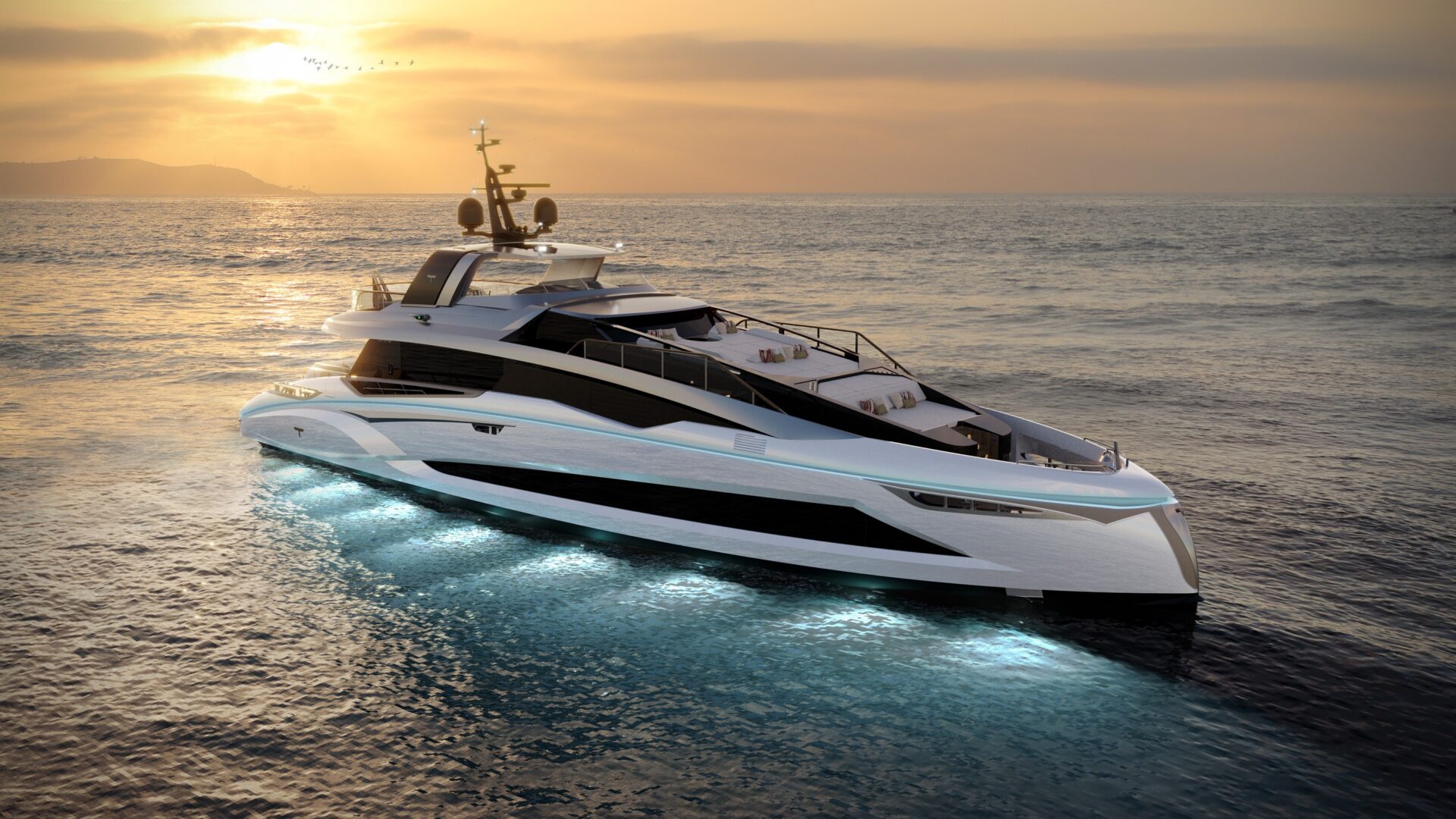The image features a breathtaking and sleek white yacht dominating the center of the frame, accentuated by stylish black windows and railings. The hull is marked by a pointed bow transitioning to a gray tip, while its flat stern hints at the possibility of jet ski storage. Illuminating the water below, bluish-green lights run along the yacht's sleek sides, casting a captivating glow. The structure includes multiple windows extending up to the bridge and the radar antennas atop. Ensuring ample space for luxury, the yacht is equipped with seating areas and lounges that might resemble beds or benches, perfect for relaxation. The background presents a mostly cloudy sky with subtle touches of orange-yellow hues from the Sun, complemented by distant hills or mountains on the far left horizon. The water around the yacht is a detailed mix of gray and blue hues, rippled yet calm, reflecting the serene ambiance. A flock of birds, possibly geese, forms a V in the sky, enhancing the natural beauty captured in this scene. This premium vessel, although not a cruise ship, suggests ample accommodation for numerous guests to enjoy a lavish experience on the open water.